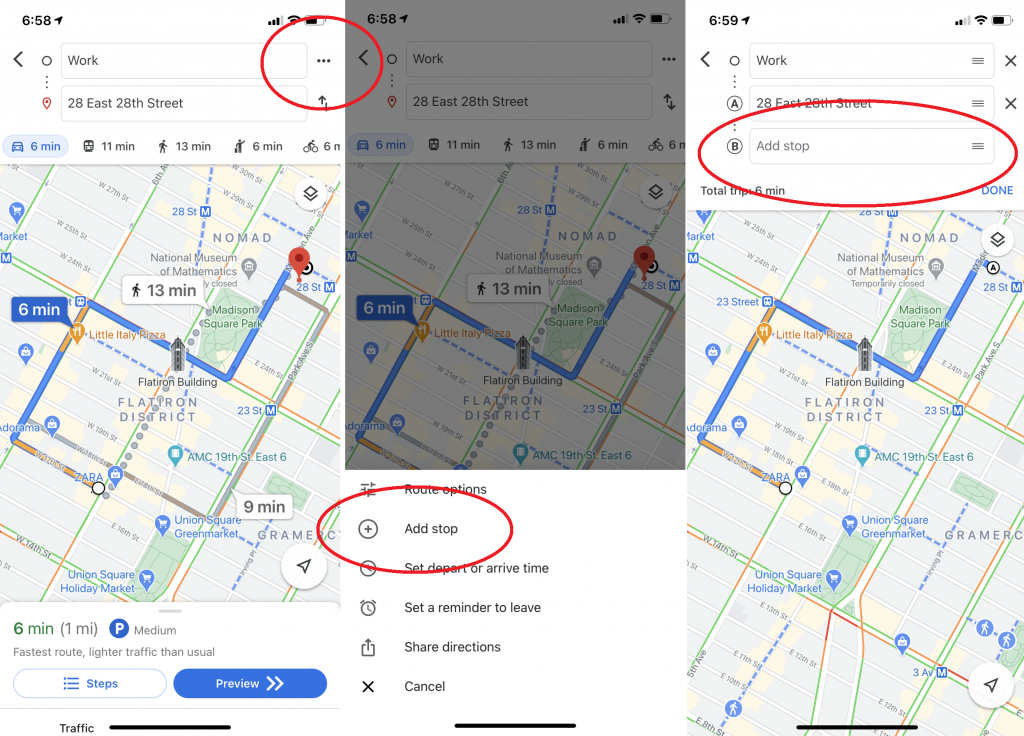The image showcases a website layout displayed in three distinct side-by-side panels.

**Panel 1:**
- Background: White
- Top Left Corner: Displays the number "658"
- Top Right Corner: Shows icons for cell signal, Wi-Fi signal, and battery life
- Left Side: An arrow pointing left, followed by a circle with three vertical dots beneath it, and a red location symbol
- Main Section: Contains a field labeled "Work" with "20 East 28th Street" beneath it
- Additional Elements: 
  - To the right of "Work" field: Three horizontal dots
  - To the right of "20 East 28th Street": A vertical double arrow
  - A red circle connecting both texts, extending into the second panel
- Travel Information: Lists durations and distances – "6 minutes, 11 minutes, 13 minutes, 6 minutes" and "6 minutes, 1 mile, 1 minute, 1 mile"
- Bottom: Options for "Steps" or "Preview"
  
**Panel 2:**
- Top: Same layout as Panel 1, including "Work" and "20 East 28th Street"
- Map: Darkened compared to the map in Panel 1
- Options Below Map: "Route options, Add stop, Set depart or arrive time, Set a reminder to leave, Share directions, Cancel"
- Highlight: "Add stop" is circled in red

**Panel 3:**
- Top: Similar layout as previous panels with "Work" and "20 East 28th Street"
- Distinguishing Feature: Includes a circle with the letter "A" and a dot sequence leading to the letter "B"
- Main Section: Focuses on an open space labeled "Add stop"
- Map: Similar to previous panels

Each panel comprehensively details a section of the website, demonstrating interactive elements, navigation, and additional functionalities available to the user.